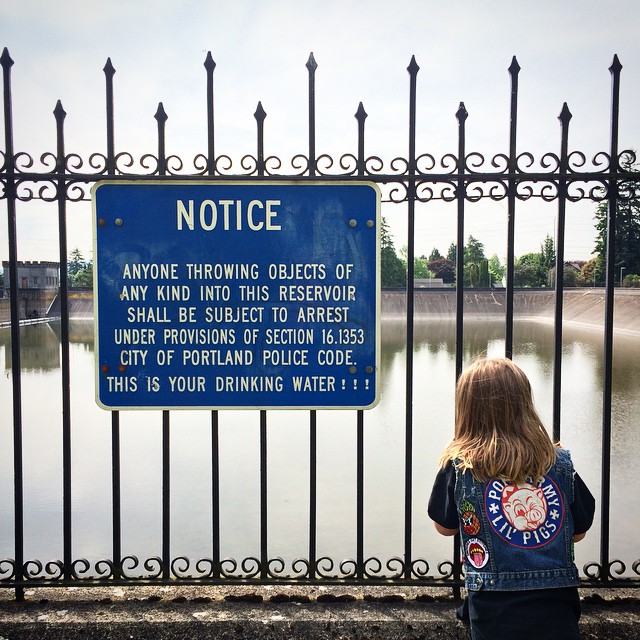In this photograph, a young girl with mid-length brown-blonde hair cascading over her blue jean vest stands peering through a black wrought iron fence at a reservoir. Her vest features a distinctive drawing of a red-nosed pig encircled on the back, accompanied by an inscription that begins with "little pigs," though the rest is obscured by her hair. The vest also has patches adorning its left side. The wrought iron fence, characterized by alternating tall and short pointed posts and decorative swirls, prominently displays a blue sign with white lettering that reads: "NOTICE, anyone throwing objects of any kind into this reservoir shall be subject to arrest under provisions of Section 16.1353, City of Portland Police Code. This is your drinking water!!!" The girl, appearing to be around seven or eight years old, holds onto the fence while gazing at the water. In the background, a house is visible among the trees, and a dam is situated in the upper left corner of the image.